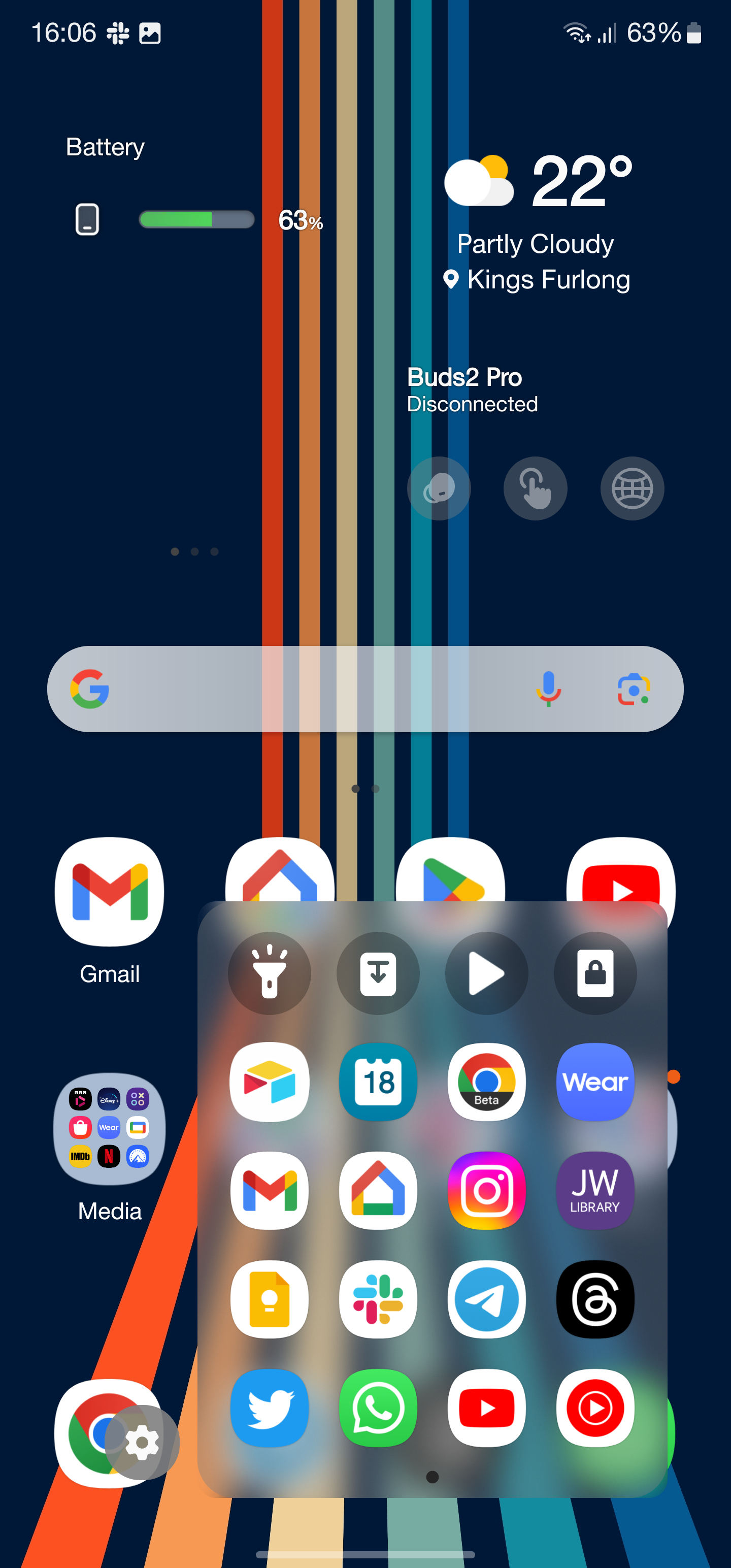A screenshot from a cell phone depicting a detailed vertical composition with various colors against a dark blue background on both the left and right sides. The central portion is adorned with a series of vertical lines in an array of colors—red, blue, dark blue, orange, dark blue, pale yellow, dark blue, blue-green, dark blue, bright blue, dark blue, and purplish blue. These lines gradually fan out towards the bottom, spreading to the left and right. At the top of the screenshot, the time is displayed as 16:06, with a battery level of 63%. The screen also shows a current temperature of 22 degrees Celsius, accompanied by a cloud icon indicating partly cloudy weather. The location specified is Kings Furlong.